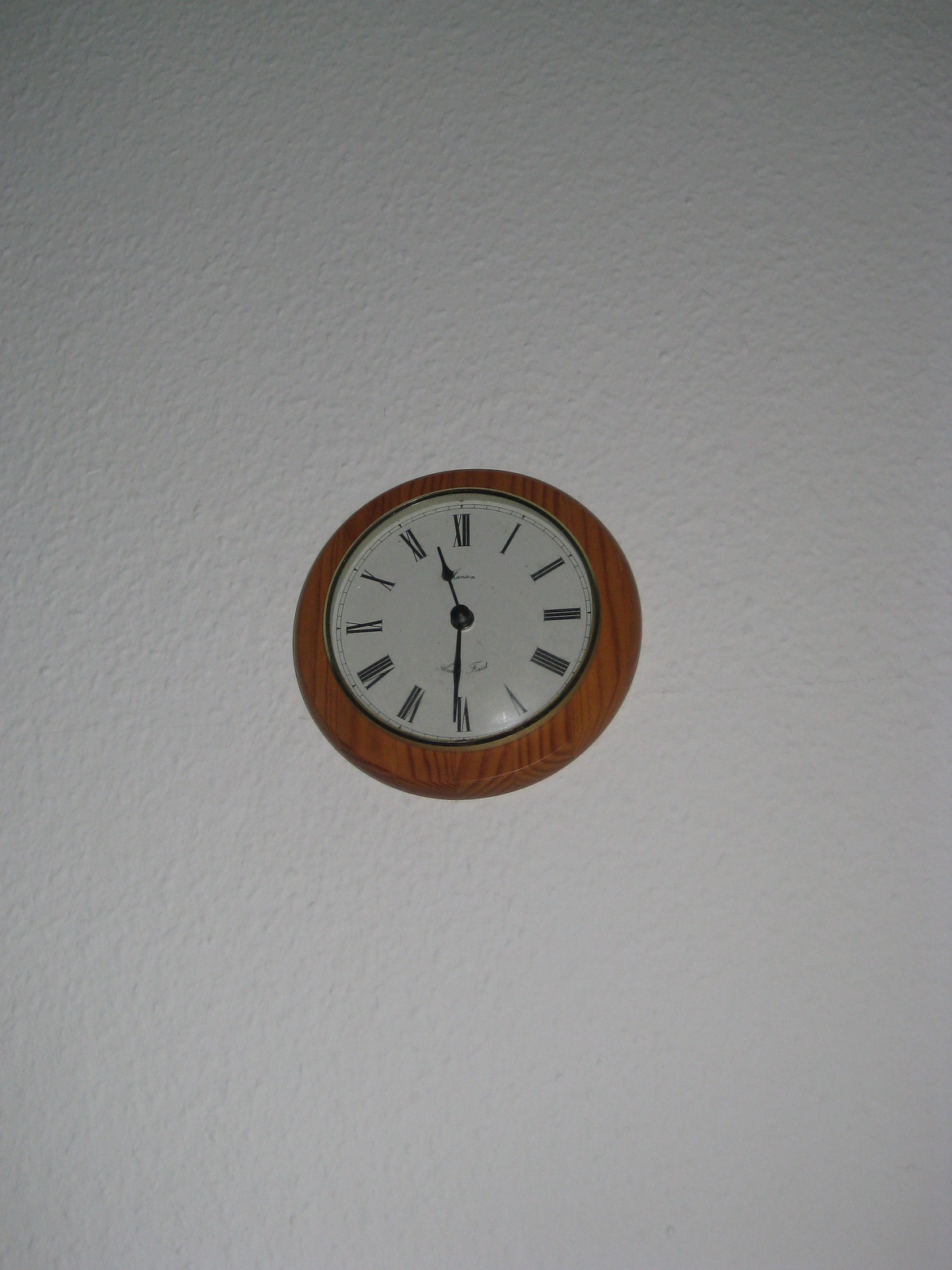The image features a wall clock centered on a textured white wall. The clock measures approximately three to four inches in diameter and has a neat, simple design. Encased in a brown, wood-stained border, the clock face boasts a clean white background adorned with thin black Roman numerals marking the hours. The numerals range from I for 1 to XII for 12. The clock hands are thin and black, with the shorter hand positioned slightly past 11 and the longer hand pointing directly at the 6, indicating a time of around 11:30 or 11:31. The brand "Cambria" is visible on the clock face, which also features small segments dividing each hour. The clock casts minimal shadow against the wall.